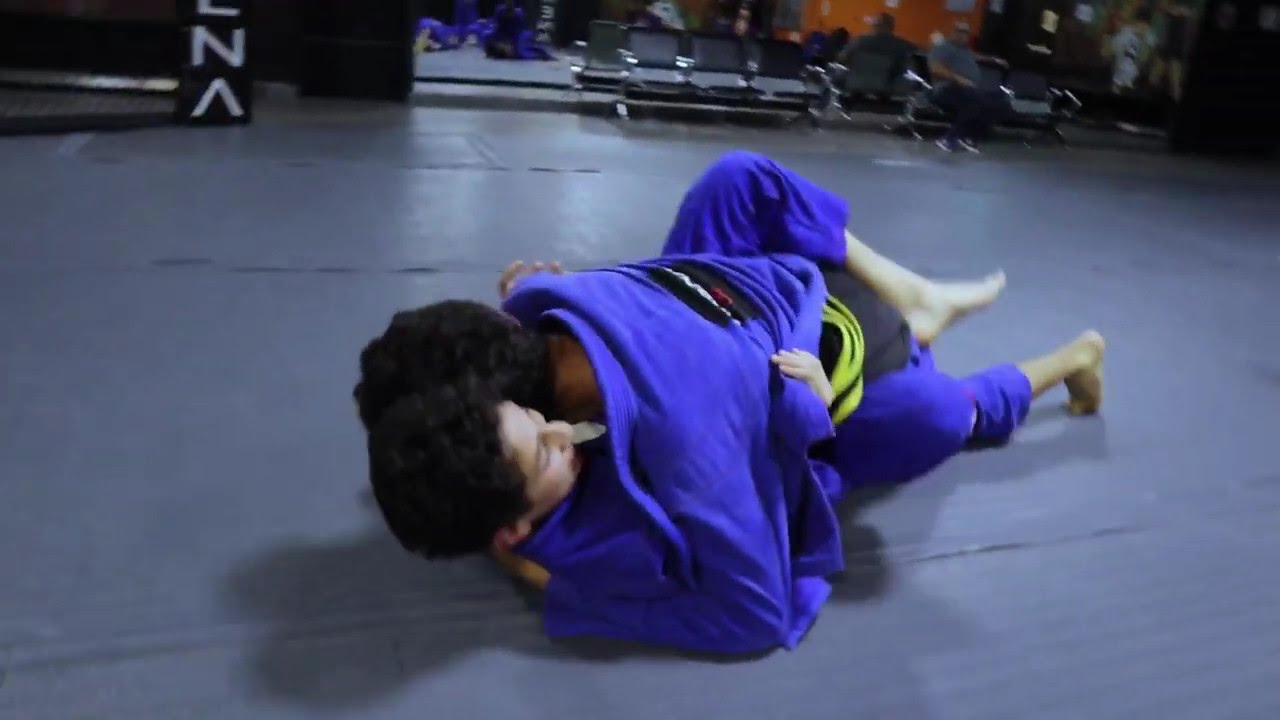This image captures a slightly blurred scene of an indoor judo match, with two players in blue uniforms on a gray mat in the center. The individuals, a man with lighter white skin and another with darker brown skin, appear to be grappling or wrestling on the ground. The setting seems to be a gym or sports hall, as indicated by the presence of an audience seated in black chairs at the top of the image. Some chairs are empty. Among the various elements, there's a mirror at the top, adding depth to the scene. The image’s color palette includes tones of gray, black, brown, tan, purple, and green. The overall impression is of a structured, yet somewhat casual, sports exhibition.